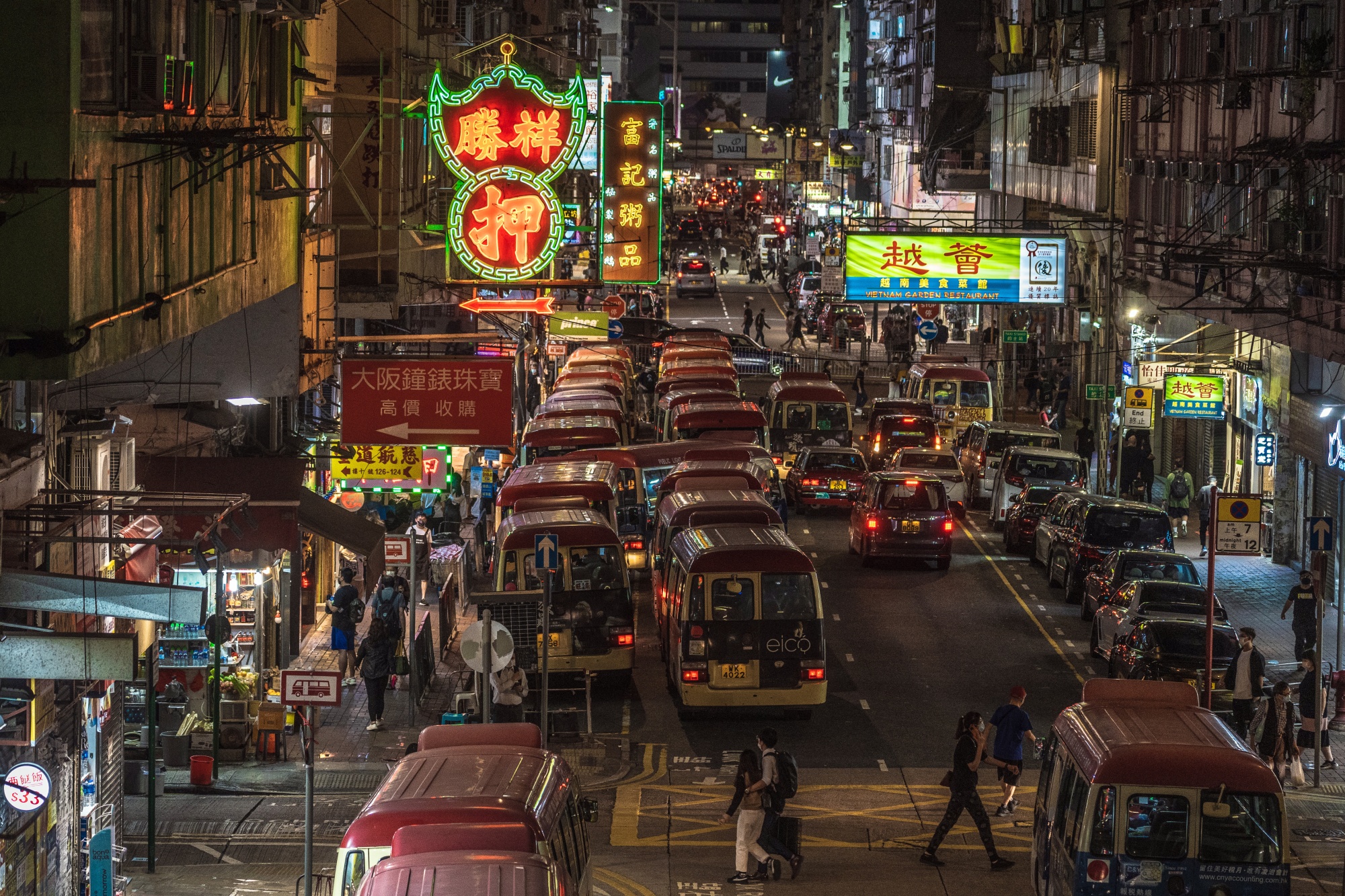The image captures a bustling night scene on a crowded street in an Asian metropolis. The street is filled with bumper-to-bumper traffic, including numerous buses with distinctive red roofs and white text spelling "ELCO". Cars are also tightly packed, their taillights glowing. Neon signs with Asian characters illuminate both sides of the street, adding vibrant color and an unmistakable cultural context. The left sidewalk is particularly crowded with pedestrians, while the right sidewalk is less populated but equally lined with brightly lit signs and little shops. High above the street, tall buildings with many illuminated windows tower over the scene, indicating an active urban environment. This busy thoroughfare, replete with people walking on crosswalks and along the sidewalks, truly epitomizes a lively Asian city by night.